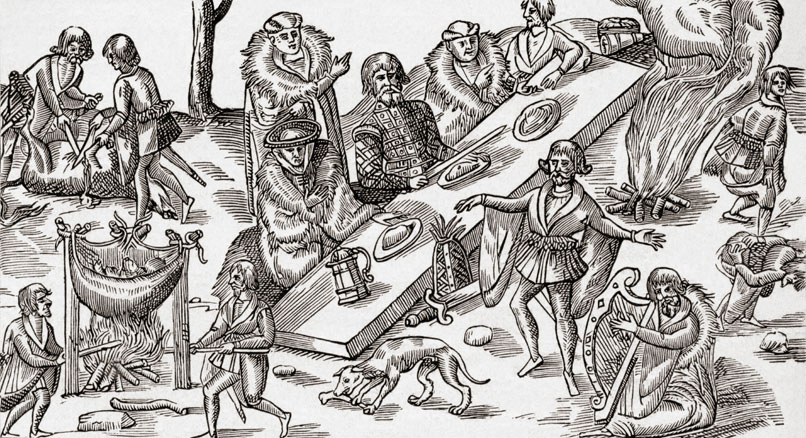The black-and-white drawing depicts a bustling scene of men engaged in various activities, with a slanted table positioned diagonally across the center. This table, which is tilted upwards toward the top right and slopes down to the ground near the bottom center, holds three dishes of food and a jug near its lower end. Four men sit on the left side of the table, facing forward, while on the right side, a man stands with his arms extended outward. They are dressed in period clothing, adding a historical context to the scene.

In the bottom left corner, two men work together, holding a stick and attending to a fire that cooks food in a pot hung between two poles. Additionally, there are details of dogs scavenging food from the ground, and a person playing a harp, enriching the scene’s ambiance. On the periphery, two other individuals appear to be butchering an animal, adding to the variety of activities depicted. The drawing captures a moment of communal effort and social gathering, with every detail contributing to the vivid portrayal of life and labor.